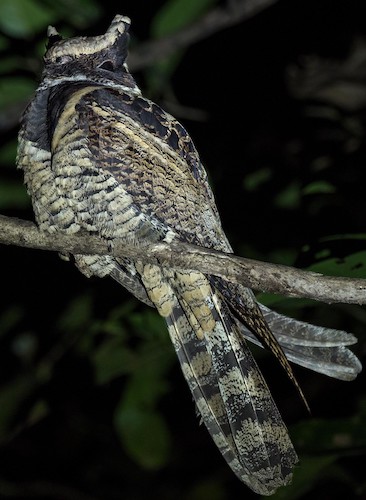The image captures a nocturnal scene featuring an owl perched on a grayish-brown branch, which is horizontally centered across the frame. The owl's back is to the viewer, with its head turned, making it impossible to see its face. Its plumage displays a mix of tan, black, and white, with distinctive tiger-stripe-like patterns on its body. The owl's ears are visible, and its long, thin tail feathers hang down below the branch. The background is predominantly black, indicating it is nighttime, with blurred green leaves and twigs adding a touch of color. The overall composition features mostly neutral tones, complemented by the green foliage and the detailed textural contrast of the owl's feathers. The photograph, likely taken by a professional, successfully keeps the owl in sharp focus while the background remains artistically blurred, though it arguably lacks the optimal face visibility. There is no discernible text within the image.